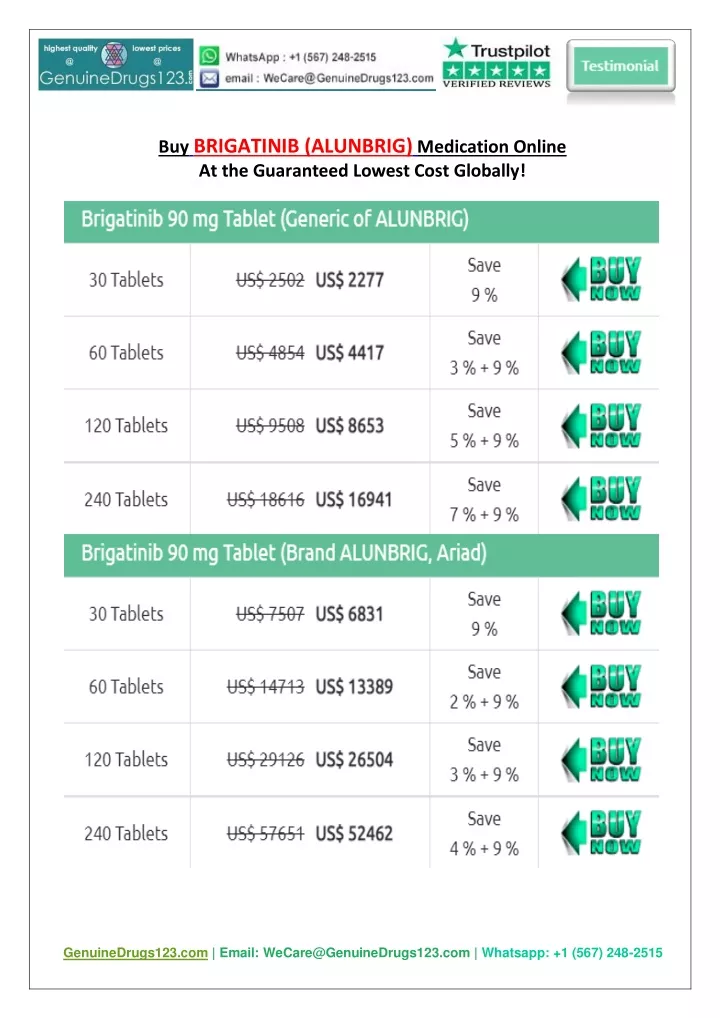The website www.genuinedrugs123.com prominently features a green rectangle with the site’s URL, where "dot-com" is creatively displayed sideways. At the top, the banner highlights "Highest Quality and Lowest Price". Adjacent to this are icons for contacting via WhatsApp and email. Additionally, the banner boasts Trustpilot Verified Reviews with a five-star rating and includes a radio button labeled "Testimonials".

Under this introductory section, the site advertises the availability of Bringitinib Allergrip medication online at the guaranteed lowest cost globally, referring to this generic drug as Allenbrick 90mg tablets. A detailed pricing table is presented next to this advertisement:

- 30 tablets for $22.77 (9% savings) - option to "Buy Now"
- 60 tablets for $44.17 (save 3% plus an additional 9%) - option to "Buy Now"
- 120 tablets for $86.53 (save 5% plus an additional 9%) - option to "Buy Now"
- 240 tablets for $166.91 (save 7% plus an additional 9%) - option to "Buy Now"

Beside this, there is information about Brigitinib 90mg tablets branded as Allenbrick Ariad, with similar purchasing options available for 30, 60, 120, and 240 tablets.